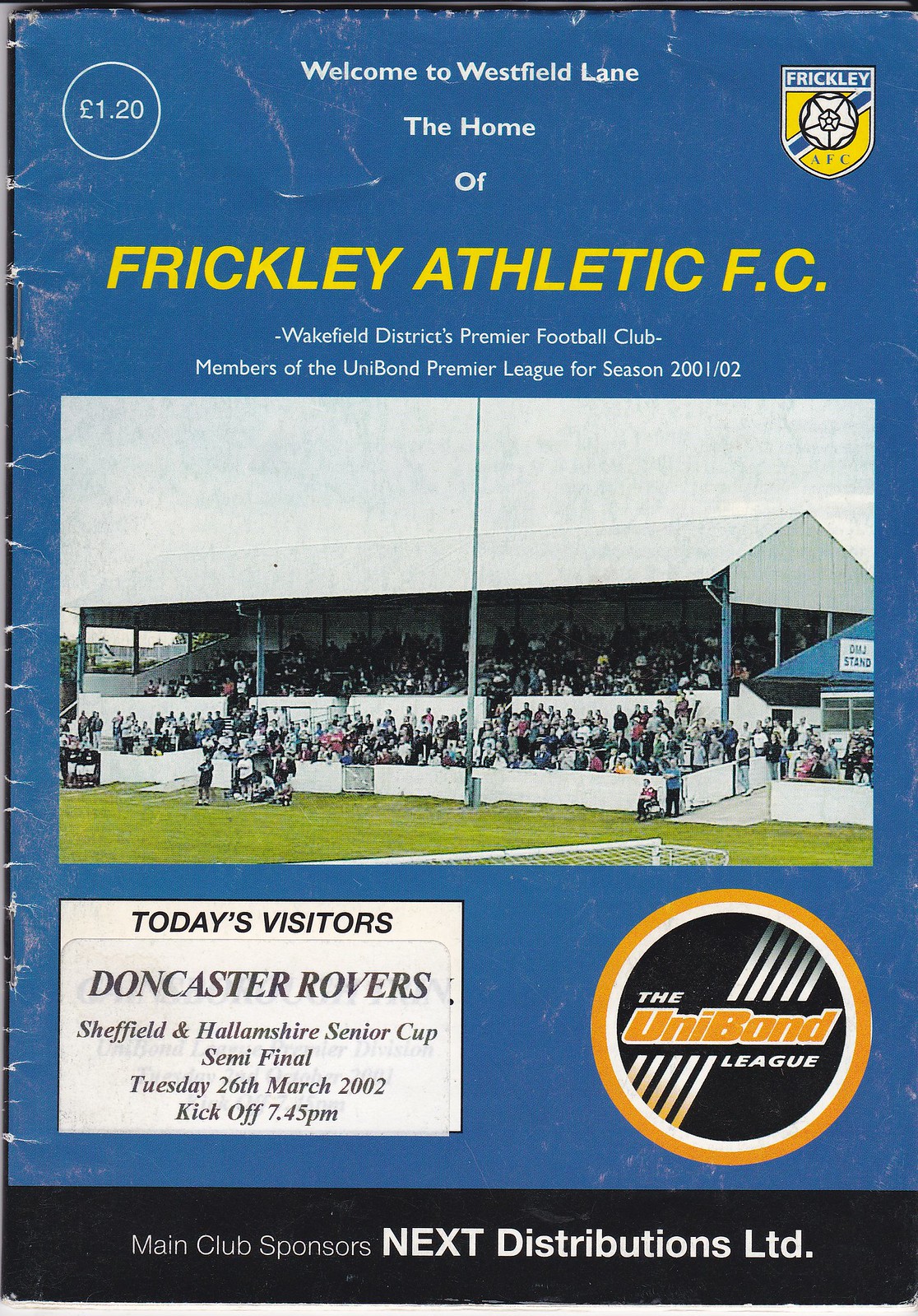This is an old, crinkled, and blue pamphlet-style magazine with a battered appearance, featuring creases and staples along the left side. The top section is marked with a price of £1.20 and announces "Welcome to Westfield Lane, home of Frickley Athletic FC, Wakefield District's Premier Football Club, members of the Unibond Premier League for season 2001-02." The Frickley AFC logo, which resembles a shield with a soccer ball and blue slash, is located in the upper right corner. Below the main heading, a large rectangular image depicts part of the football pitch, visible green grass, and a basic stadium structure with a covered grandstand. The seating area has a white roof with some side coverings, but remains mostly open. Below the image, text reads, "Today's Visitors, Doncaster Rovers, Sheffield, and Hallamshire Senior Cup semi-final, Tuesday 26th March 2002, kickoff 7.45pm." On the bottom-right side of this section is an orange circle with the text "The Unibond League," surrounded by circular dash marks. At the bottom, a black border announces, "Main Club Sponsors, Next Distributions Limited."